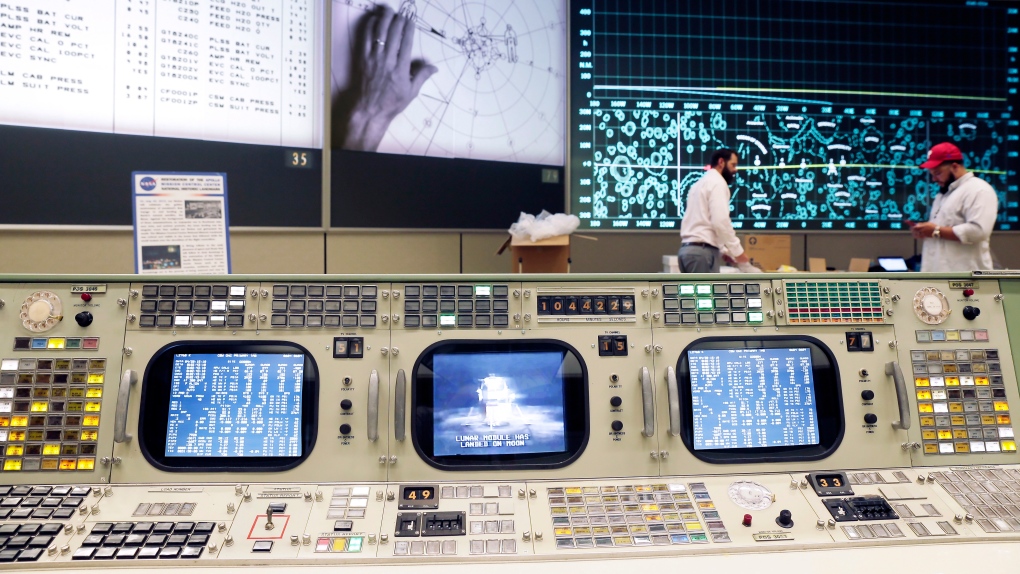This image captures the bustling atmosphere of a NASA mission control room. Dominating the foreground is a large control panel filled with an array of buttons, switches, and three computer screens, each displaying various streams of data and images, including potential ship trajectories and graphs. Two bearded men, both dressed in white shirts with one sporting a red hat, are actively engaged in work, inspecting boxes or equipment. Behind them, a large digital display stretches across the wall, showcasing detailed information and proudly bearing the NASA logo in its top left corner. The high-tech yet somewhat vintage setup underscores the room's critical role in managing and monitoring complex missions.